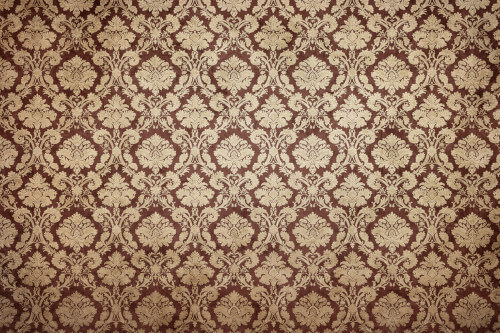This image depicts a detailed, intricately designed pattern reminiscent of traditional wallpaper or a decorative rug. Dominated by deep, earthy tones, the pattern features a backdrop in a rich, rusty brown hue enhanced by elements of tan and dark red. At its core, there's a repeating symmetrical design that extends seamlessly from one edge to another. This pattern is characterized by abstract motifs that resemble treetops or shrubs, crafted in prominent beige and gold hues. Interwoven in this design are central roundish shapes that could be interpreted as faces or floral elements, surrounded by a trellis-like structure. The overall effect is a harmonious, upscale floral motif that exudes symmetry and elegance.